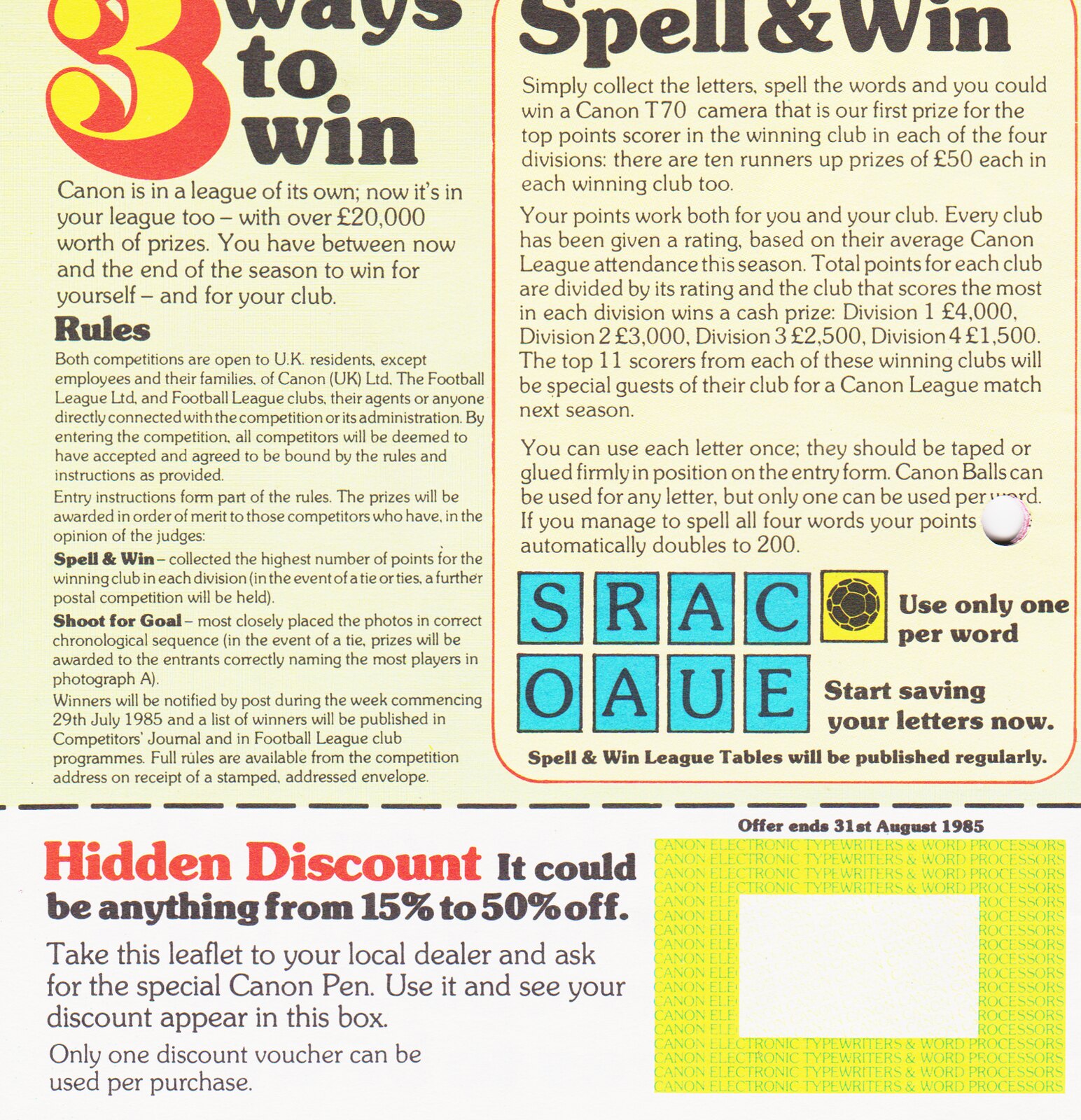This image appears to be a magazine or newspaper insert featuring a contest and coupon details. The top portion of the page has a light yellowish background, and the content is divided into two text columns. The left column prominently displays a large number three in yellow and red, followed by the text "ways to win" in black font. The text continues with "Canon is in a league of its own. Now, it's in your league too, with over £20,000 worth of prizes. You have between now and the end of the season to win for yourself and for your club." Beneath this, the rules specify that both competitions are open to UK residents, except for employees and their families of Canon UK Limited, the Football League Limited, and Football League Clubs. Additional rules and text are also provided.

On the right column, the top section instructs on the "Spell and Win" contest, urging participants to collect letters and spell words for a chance to win a Canon T70 camera. This is the first prize for the top point scorer in the winning club in each of the four divisions. There's extensive text in both columns outlining further details. The bottom right highlights that the offer ends on 31st August 1985. Meanwhile, the bottom left details a "hidden discount" offer, which could range from 15% to 50% off, potentially revealed by peeling off a yellow box.